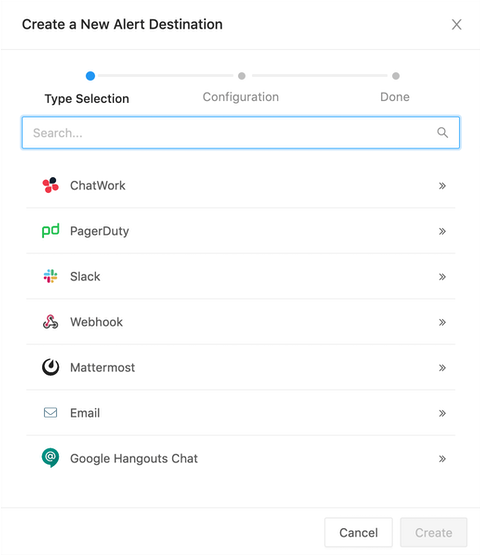The image features a clean, white background populated by various texts and logos centrally arranged. At the top left, there is a bold black text reading "Create a New Alert Destination." On the far right, there is a light gray 'X' mark, which is accompanied below by a thin, light gray line. Under this line, there is a long horizontal, light gray bar stretching across the center.

Starting from the left side of the bar, there is a small blue dot. Below this blue dot, black text reads "Type Selection." Directly under this, there is a wide rectangular white box bordered in blue with light gray placeholder text inside that says "Search."

Adjacent to the left end of the horizontal line in the center, there’s a light gray button labeled with the black text "Configuration." To the right of this button is another light gray button, beneath which is the text "Done."

Below the search bar on the left side, there is a vertical list of black texts paired with distinct logos. The first item reads "Chatwork" beside which are four colored dots arranged in a diamond shape. Underneath this is "PagerDuty" with an accompanying green "PD" logo. Following that, "Slack" is listed with its characteristic multi-colored dot logo to its left. Next, "Webhook" is indicated beside an abstract triangular icon. Below it, "Mattermost" is present with a black circular logo. Further down, "Email" appears next to a blue postcard icon. At the bottom, "Google Hangouts Chat" is visible with a dark green circular logo to its left.